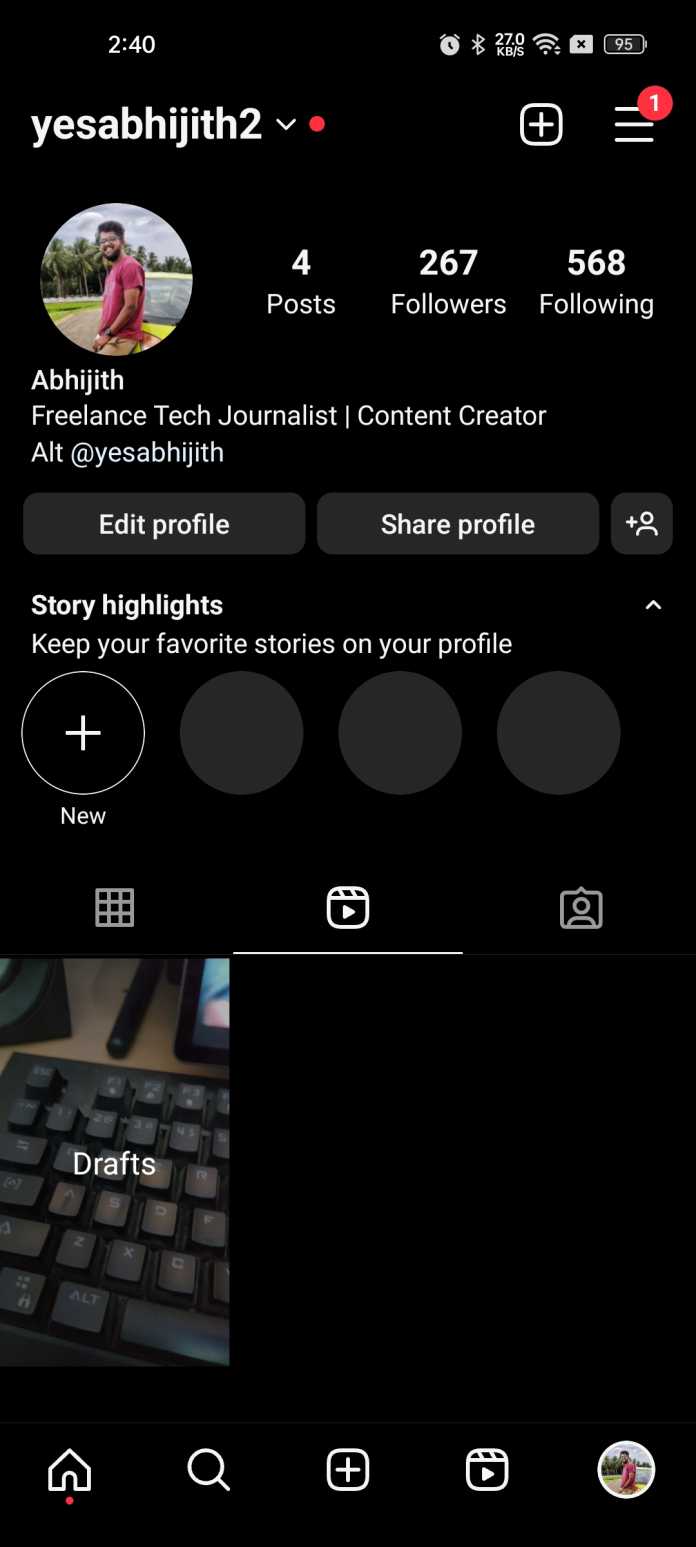A detailed screenshot from a smartphone display captures various interface elements and a profile of a social media user. At the top left corner, the time reads 20:40, likely in military time, accompanied by an alarm icon, a Bluetooth icon, and an internet speed indicator showing 27.0 kbps. The Wi-Fi symbol illustrates full signal strength, while a SIM card icon with a black X suggests missing or unavailable cellular service. On the top right, the battery icon shows 95% charge.

The central focus of the screenshot is a profile featuring a portrait of a muscular man with short black hair and a long black beard. He is wearing a red t-shirt with white text and tan khakis, sitting on a yellow car amidst a backdrop of dark green trees and grass, beneath dark grey and white storm clouds. Above his portrait, in bold white text, is his username: "YESABHIJITH2," with a dropdown arrow and a red circle. To the right of the portrait, details in white text indicate he has made 4 posts, has 267 followers, and is following 568 accounts.

Beneath the portrait, the name "ABHIJITH" is followed by the descriptors "freelance tech journalist" and "content creator" separated by a line. A mention, "@yesABHIJITH," is indicated for ALT. Two clickable buttons are displayed below: a black rectangle with "Edit Profile" in bold white text and a white rectangle with "Share Profile" in bold black text. A third option is a dark black square with the silhouette of a person and a plus sign, suggesting the option to follow this profile.

Below these buttons, in bold white text, "Story Highlights" is shown with a subtler text urging to "keep your favorite stories on your profile." There are three empty black circles and an additional circle on the far left with a white cross through it, bordered in white, labeled "New."

Towards the bottom, a "drafts" section displays a close-up image of a black keyboard with white keys, indicating it is a saved draft.